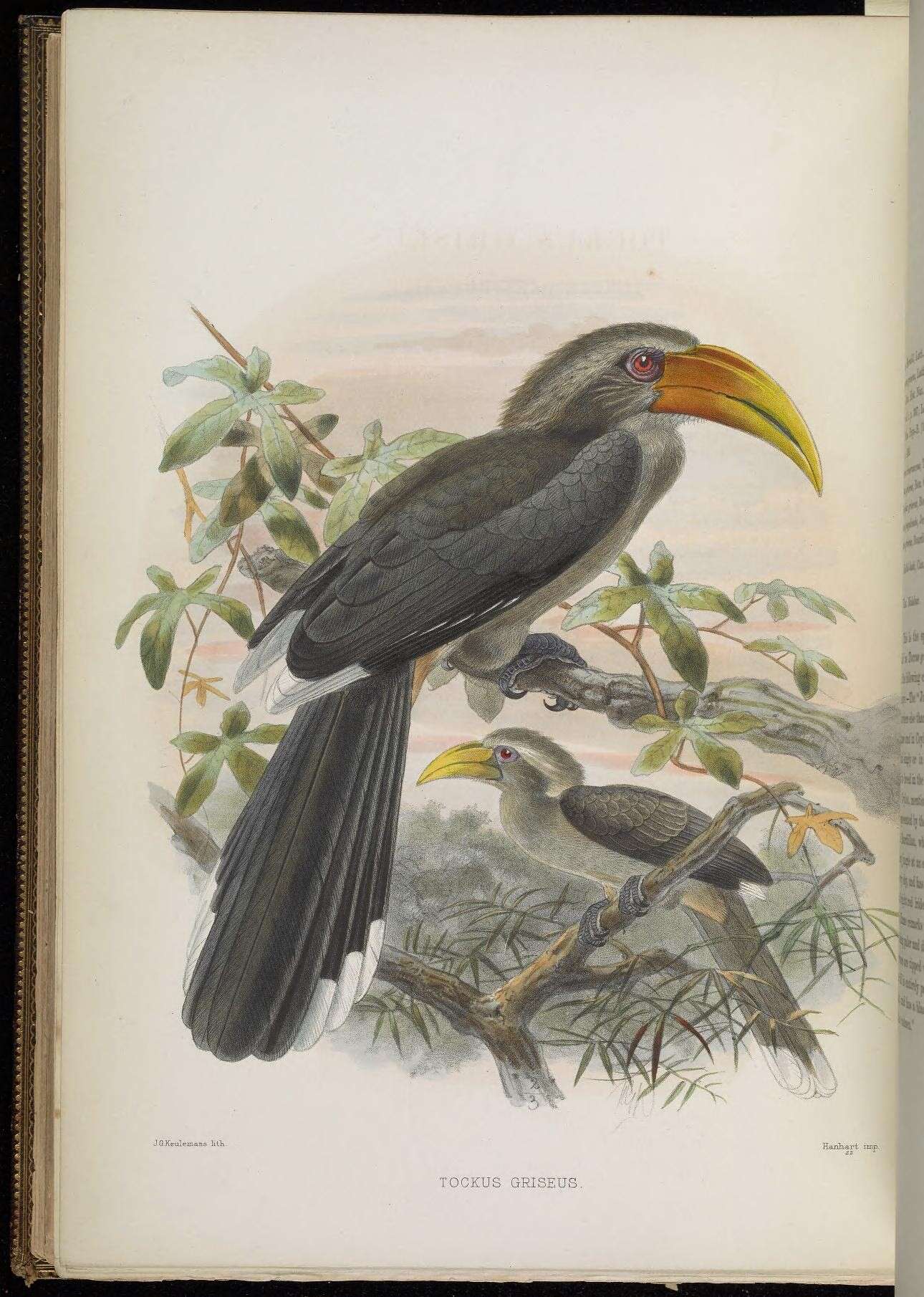A detailed illustration from an old hardcover science book appears on the left-hand page, depicting two birds identified as "Tachysclerosis" against a white background. The image showcases watercolor or ink drawings featuring toucan-like birds with distinctive long tails. Both birds display black and white tail feathers, black wings with white tips, and yellowish-orange beaks. The top bird has a reddish hue to its beak, grayish-brown underbelly, and brown eyes. In contrast, the smaller bird at the bottom has a lighter-colored chest and an all-yellow beak. The birds are perched on tree branches adorned with mixed green leaves, including thicker leaves at the top and thinner ones at the bottom. The surrounding text, indicating "Tochis griseus," suggests a scientific, encyclopedic context. The right-hand page, visible in part, features only black text on a white background, further emphasizing the detailed ornithological illustration on the left.